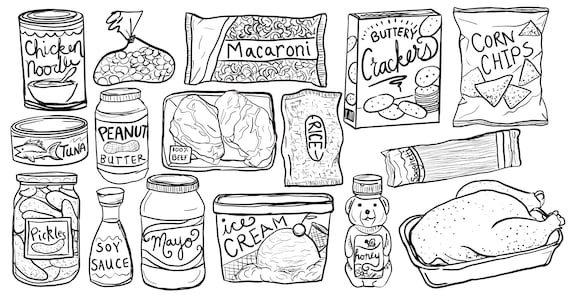The image is a seamless collection of black-and-white doodle-style drawings of various staple food items, all on a white background. Each item is clearly labeled in the center with basic descriptions, devoid of specific brand names. From left to right, top to bottom, the foods depicted include a can labeled "chicken noodle soup," a plastic bag that likely contains peanuts, a bag of macaroni that says "macaroni," a box marked "buttery crackers," and a bag labeled "corn chips." Below these, there's a can of tuna illustrated with a fish, a jar of peanut butter, a package indicating "100% beef," a pack of rice, and a pack of spaghetti noodles. The final row features a jar of pickles, a container of ice cream, a jar of mayo, soy sauce, a bear-shaped bottle of honey, and a pan with either a chicken or turkey. The simplicity of the black-and-white drawings makes each food item easily recognizable.